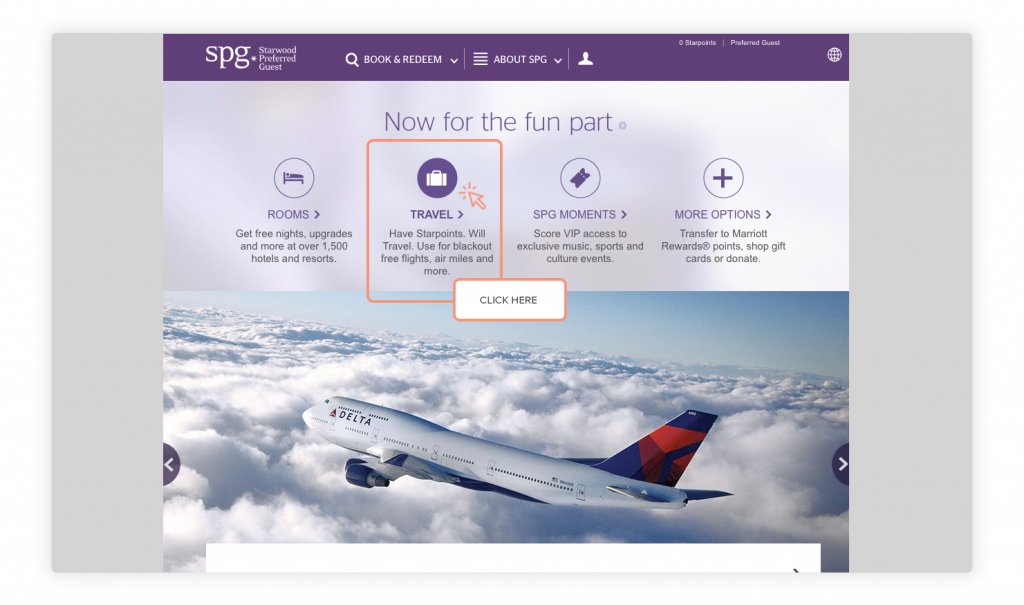The home page of the Starwood Preferred Guest (SPG) website features a sleek navigation bar at the top with a deep purple background. Prominently displayed on this bar is the SPG logo, accompanied by small text. To the right, there are 'Book' and 'Redeem' buttons, which appear to trigger a dropdown menu with further options upon hovering.

The navigation bar also includes a section labeled 'About SPG,' highlighted by an icon resembling a man's silhouette, likely serving as a profile or member information link. 

Below this bar, the main content area showcases a stunning photograph of a Delta commercial airliner soaring above the clouds, alongside the caption, "Not for the fun part." 

Further navigational options such as 'Rooms,' 'Travel,' 'SPG Moments,' and more are listed below the main image. A highlighted box surrounds the 'Travel' link, with an accompanying annotation indicating "click here," suggesting that the image has been edited to guide users on how to navigate the site. The design employs a pleasing color palette of whites and purples, giving the page a harmonious and user-friendly aesthetic.